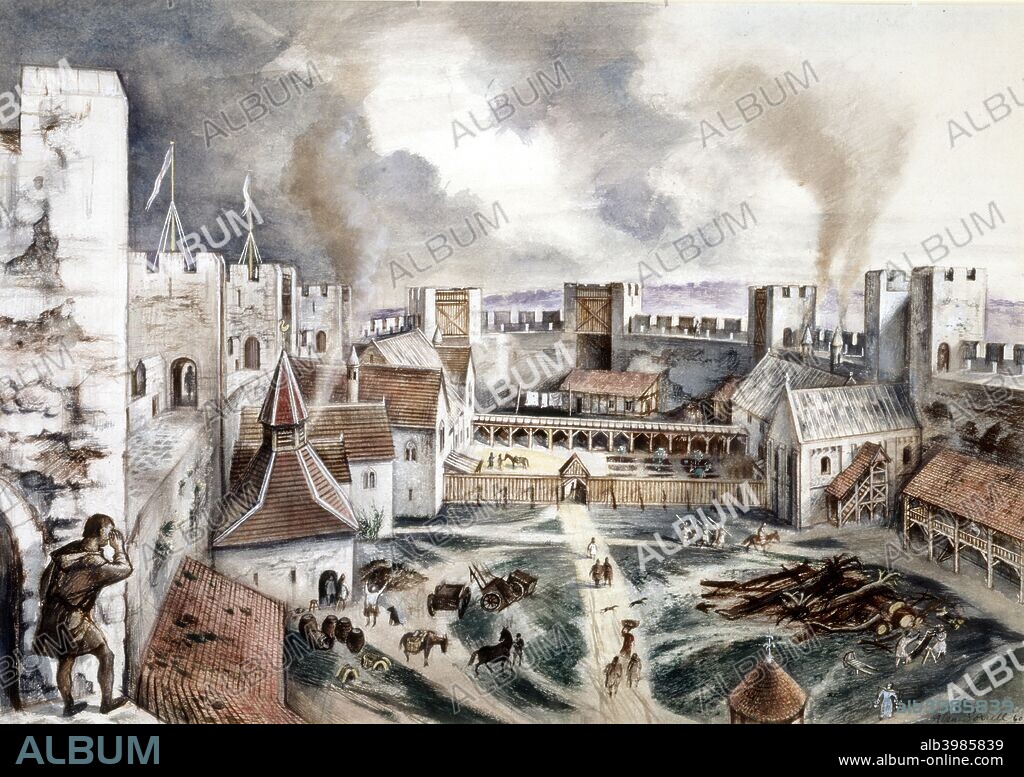The illustration depicts a medieval village enclosed within fortress walls, characterized by a blend of structures such as churches, farming buildings, and village houses. The scene reveals a prominent figure stationed on the lower left wall, vigilantly observing the courtyard below for potential threats. The foreground shows villagers and domesticated animals, including horses and mules, moving about the courtyard, which is bordered by old, square-topped buildings. The sky is ominously gray, interspersed with smoky plumes, suggesting that the village may be under siege. The colors utilized are predominantly off-whites, grays, brown, red-brick tones, and patches of light green grass. A repeating watermark of "album" is superimposed across the illustration, and the lower right corner prominently features a black border with the URL www.album-online.com.